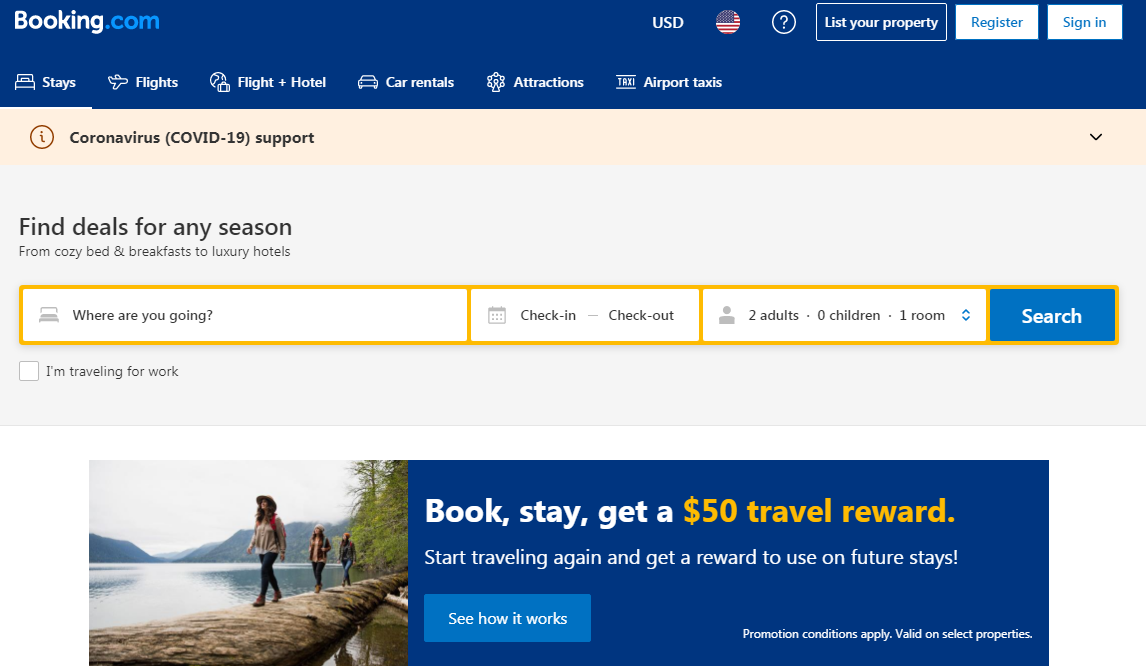This image showcases the homepage of the Booking.com website. The top of the page features a blue border with the Booking.com logo prominently displayed on the left side; "booking" is in white text, and ".com" is in blue. To the right of the logo, the header includes options such as the currency selector "USD," accompanied by an American flag, a help button represented by a question mark inside a circle, buttons for "List your property," "Register," and "Sign in."

In the lower left corner of the blue border, there are navigation links labeled "Stays," "Flights," "Flight + Hotel," "Car Rentals," "Attractions," and "Airport Taxis." Just beneath this blue border, a beige or peach-colored dropdown box offers "Coronavirus (COVID-19) support."

Below it, a light gray box encourages users to "Find deals for any season—from cozy bed and breakfasts to luxury hotels." Following this, there is a prominent search box prompting users with "Where are you going?" alongside fields to select "Check-in" and "Check-out" dates, the number of "Adults," "Children," and "Rooms" required, and a "Search" button to submit these details.

Additionally, there is a checkbox option labeled "I'm traveling for work." At the very bottom of the screen, a banner invites users to "Book stays, get a $50 travel reward. Start traveling again and get a reward to use on future stays," along with a button directing users to "See how it works."